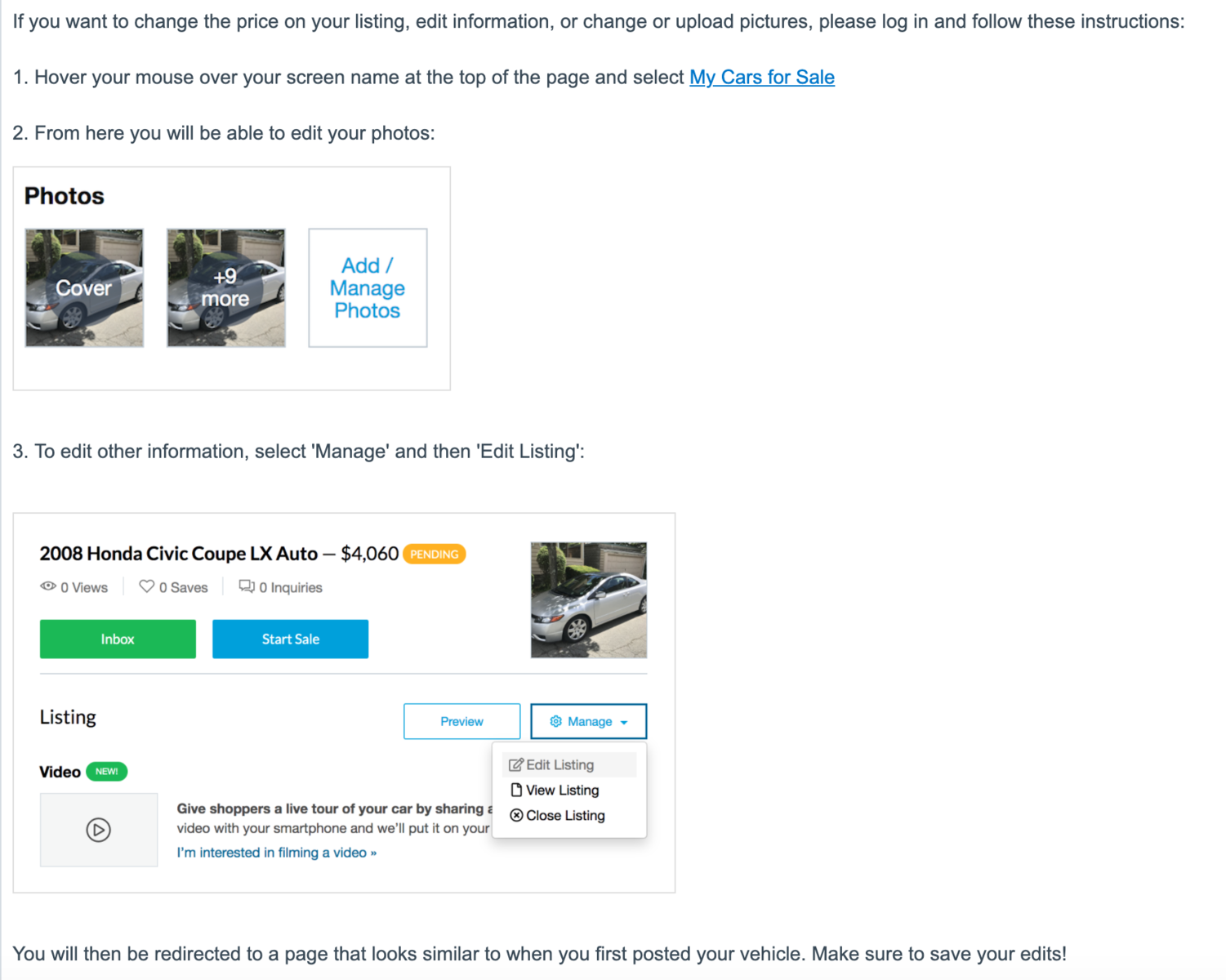This image is a screenshot of an online car sale listing for a 2008 Honda Civic Coupe LX Automatic, priced at $4,060. On the left side of the screenshot, detailed information about the car is displayed, including the option to view nine additional photos, though only one image of the car is currently visible. The bottom of the screenshot features two buttons labeled "Inbox" and "Start Sale." The right side of the image is predominantly an empty space. A sentence at the bottom advises users that after making edits, they will be redirected to a familiar page, similar to when they first posted their vehicle, and reminds them to save any changes. The page lacks any identifying website name or URL, suggesting this is merely a screenshot of the listing's interface.